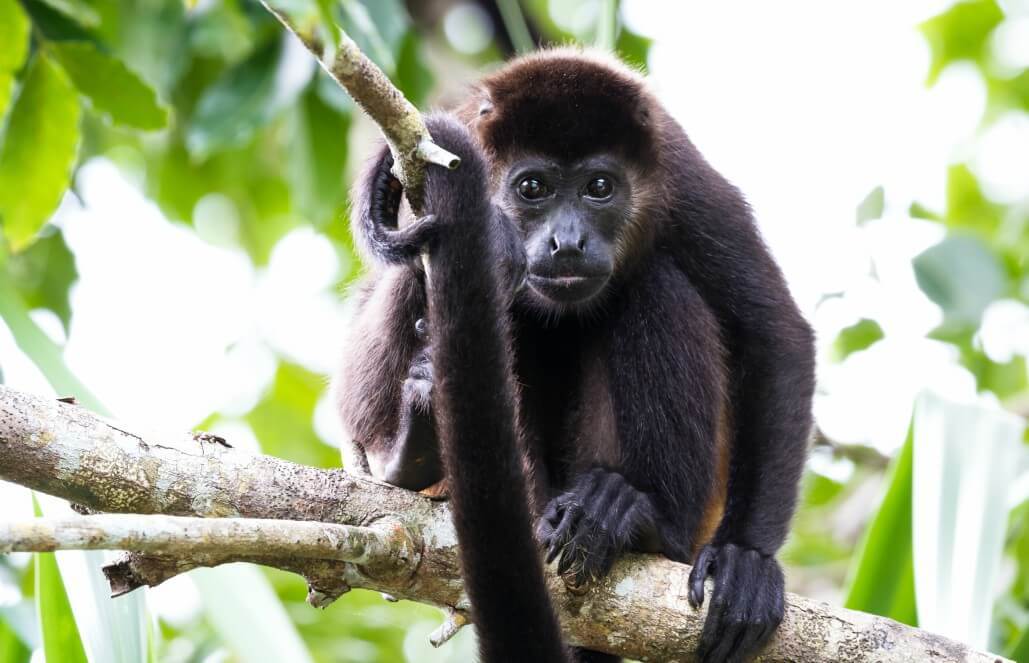In this professional outdoor photograph, an adorable baby monkey is the central focus, seated on a sturdy, wide tree branch that diagonally rises from the lower right to the middle left of the image. The monkey, covered in dark, black, and brown fur, is crouched with its hind legs bent at the knees and its shoulders drooped forward. It gazes directly into the camera with bright, wide black eyes that reflect the sunlight, exuding a sense of curiosity.

The scene is set in a sunlit, tropical forest environment, with a blurred background filled with bright green leaves and a washed-out sky, indicating daylight. The monkey's left arm extends downward, holding the branch, while its right arm bends at the elbow, seemingly holding something near its face, partly obscured by its incredibly long tail. This prehensile tail wraps under the branch and curves up in front of the monkey's face. Adding to its charm, the monkey's face is a mix of darker hues with a lighter gray muzzle and black eyes, giving it an endearing and inquisitive expression.